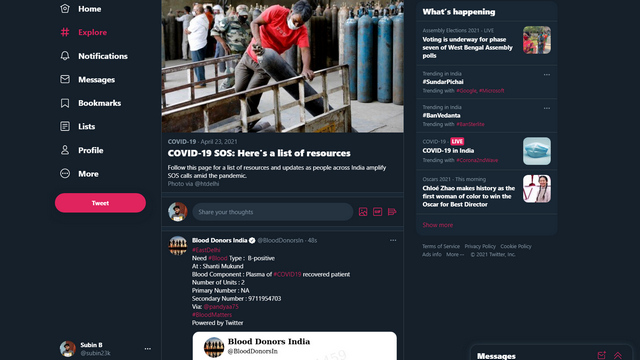This is a screenshot of a Twitter interface in dark mode, characterized by its black background. It features three distinct sections: 

1. **Left Pane:**
   - This panel displays the main navigation menu of Twitter, which includes icons and text for 'Home,' 'Explore' (represented by a hashtag), 'Notifications,' 'Messages,' 'Bookmarks,' 'Lists,' 'Profile,' and 'More.' 
   - At the bottom of the menu, there is a prominent pink button labeled 'Tweet.'

2. **Middle Pane:**
   - Dominating the center of the screenshot is an article titled "COVID-19 SOS: Here's a list of resources," posted on April 23, 2021.
   - The article is accompanied by an image of a man wearing a mask and dragging an oxygen tank in what appears to be a factory setting. Numerous oxygen tanks are grouped together in the background, highlighting the critical need for oxygen amid the COVID-19 crisis.
   - Below the article, there is a response from 'Blood Donors India,' which provides detailed information regarding blood types and contact numbers, including both primary and secondary numbers for potential donors.

3. **Right Pane:**
   - The 'What's happening' section displays a list of trending news and topics on Twitter, which are likely related to the central theme of the article in the middle pane. This section keeps users updated with the latest updates and discussions surrounding COVID-19 and other current events.

This well-organized layout provides a snapshot of the resources, responses, and ongoing conversations about the COVID-19 pandemic on Twitter.